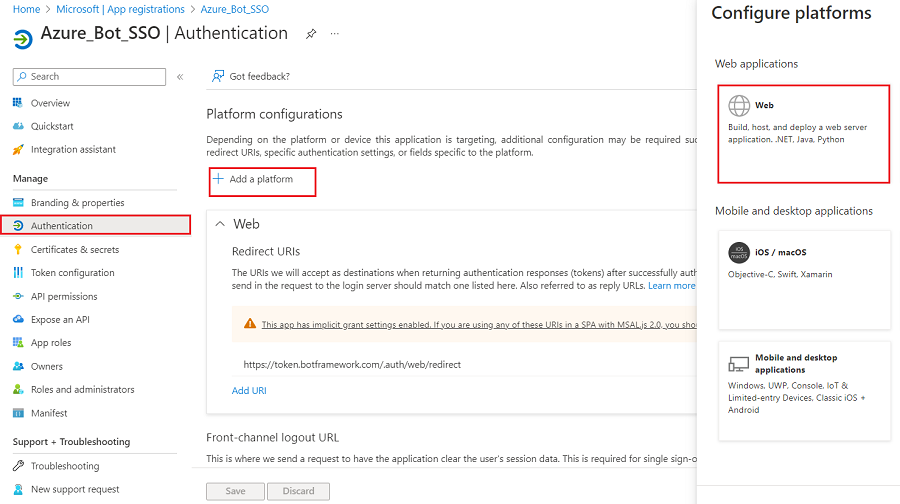A detailed and cleaned-up caption for the described image might look like this:

---

The screenshot depicts a webpage from the Microsoft Azure portal focused on Azure Bot Single Sign-On (SSO) authentication. At the top, a navigation bar features options such as "Home," "Microsoft," "App Registrations," and "Azure Bot SSO." Below this, a larger heading displays "Azure Bot SSO Authentication" prominently, accompanied by a pin icon and three dots for additional options.

On the left sidebar, which includes a search bar at the top, there are several menu items with accompanying icons: "Overview," "Quick Start," "Integration Assistant," followed by a section titled "Manage" in bold black font. Under the "Manage" section, options like "Branding and Properties" are listed, with the "Authentication" option currently selected.

To the right of the sidebar, the main content area displays a page titled "Platform Configurations." This section includes a note indicating that additional configuration might be necessary depending on the targeted platforms. A prominent red "Add a platform" button with a plus symbol sits below this note. Further down, there are fields for "Web Redirect URLs" and "Front Channel Logout URL," among other settings.

In the same content area, a section indicating feedback collection is visible, as well as detailed instructions about configuring platforms, with "Web" being the currently selected option. This suggests that the user is in the process of setting up web platform configurations for Azure Bot SSO.

---